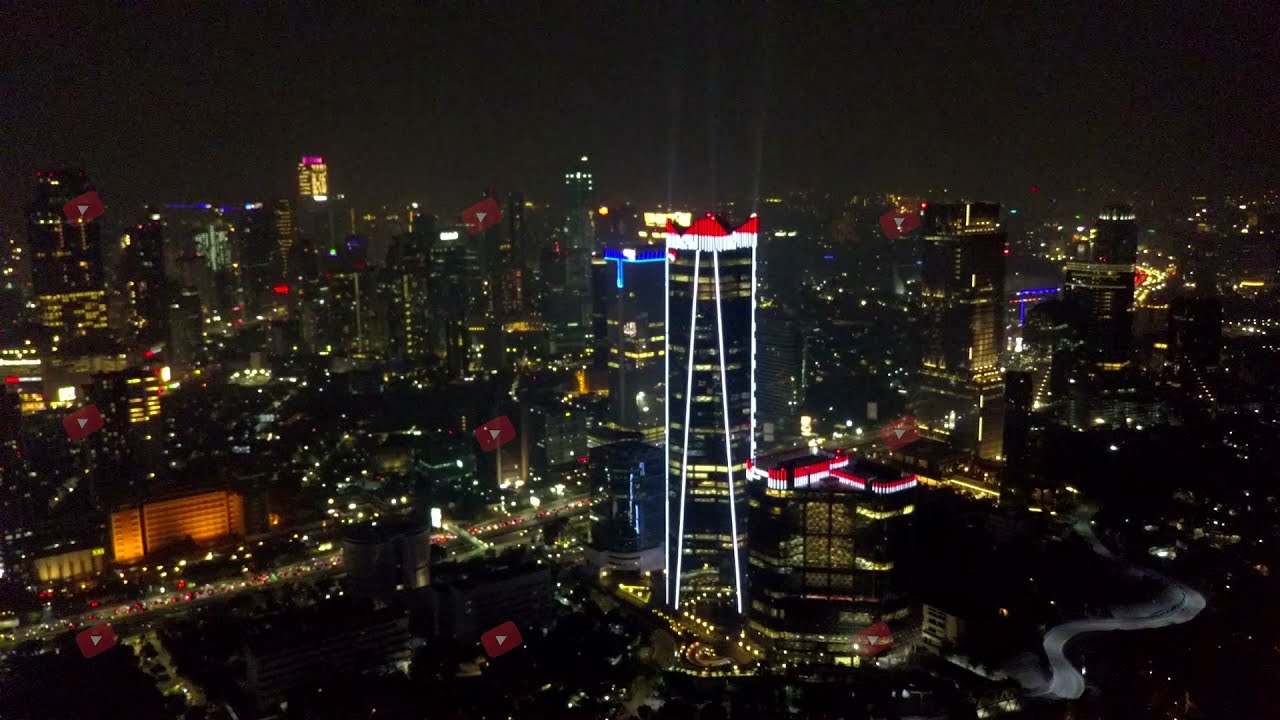This image captures a vibrant cityscape at night from an elevated viewpoint. The city below is alive with glowing artificial lights illuminating numerous multi-story buildings and towering skyscrapers. The streets, filled with shimmering vehicle headlights, weave through the urban landscape. Dominating the scene is a central skyscraper adorned with striking red peaks at its top, from which beams of light ascend into the dark sky. This building features white lights running vertically along its edges and around it, adding to its grandeur. To the right, a shorter building echoes this design with a red-topped structure and white-lit sections. The city is a tapestry of color, with smatterings of yellow, red, and pink lights providing a lively and colorful nighttime tableau.